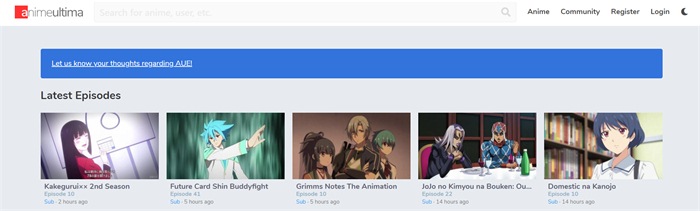This image is a cropped screenshot of the website "Anime Ultima," focusing on the top section. On the left side, the Anime Ultima logo is visible, beside which lies a search bar labeled "search for anime, user, etc." with an accompanying magnifying glass icon. Adjacent to the search bar are four navigation tabs: "Anime," "Community," "Register," and "Login," with a moon icon next to the "Login" tab. Beneath this navigation bar, a blue banner displays a white-font message that reads, "Let us know your thoughts regarding ALJE," although the acronym at the end is slightly difficult to discern clearly. Below this banner, in bold black font, is a header labeled "Latest Episodes." Under this heading, five different anime thumbnails are displayed, each representing a recently uploaded episode. The titles and details of these episodes are as follows:

1. **Kakegurui xx - Second Season, Episode 10**: Subbed, uploaded 2 hours ago.
2. **Future Card Shin Buddyfight, Episode 41**: Subbed, uploaded 5 hours ago.
3. **Grimms Notes The Animation**: Subbed.
4. **JoJo no Kimyou na Bouken**: Subbed.
5. **Domestic na Kanojo**: Subbed.

This screenshot highlights the most recent additions to their anime library, aiming to keep users updated with the latest episodes available on the site.